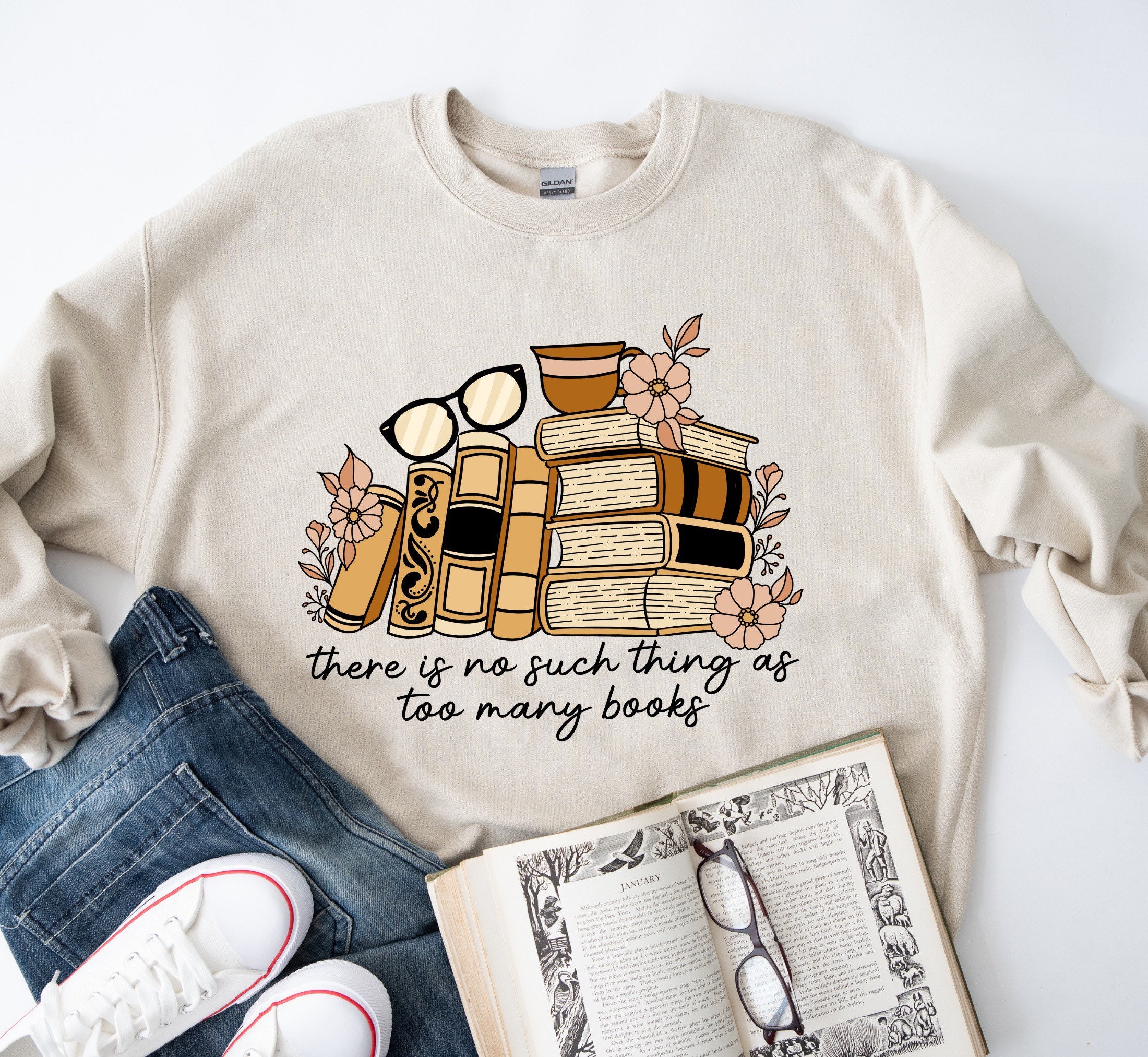This is a meticulously staged, square, full-color indoor photograph showcasing a neatly arranged flat lay. The background is a clean, white countertop. In the upper left corner, the light source creates a washed-out effect. The main focus is a light tan, long-sleeved shirt with pronounced crinkles in its fabric. The shirt prominently displays a whimsical graphic of stacked and leaning books, adorned with a coffee cup and eyeglasses, surrounded by delicate flowers. The text on the shirt reads, "There is no such thing as too many books." 

In the lower left corner, a pair of white tennis shoes with red trim rests alongside blue jeans. Dominating the bottom center is an intricately decorated open book, displaying the word "January" with a pair of folded black-framed glasses nestled in its seam. The well-composed layout casts subtle shadows, adding depth to the scene.